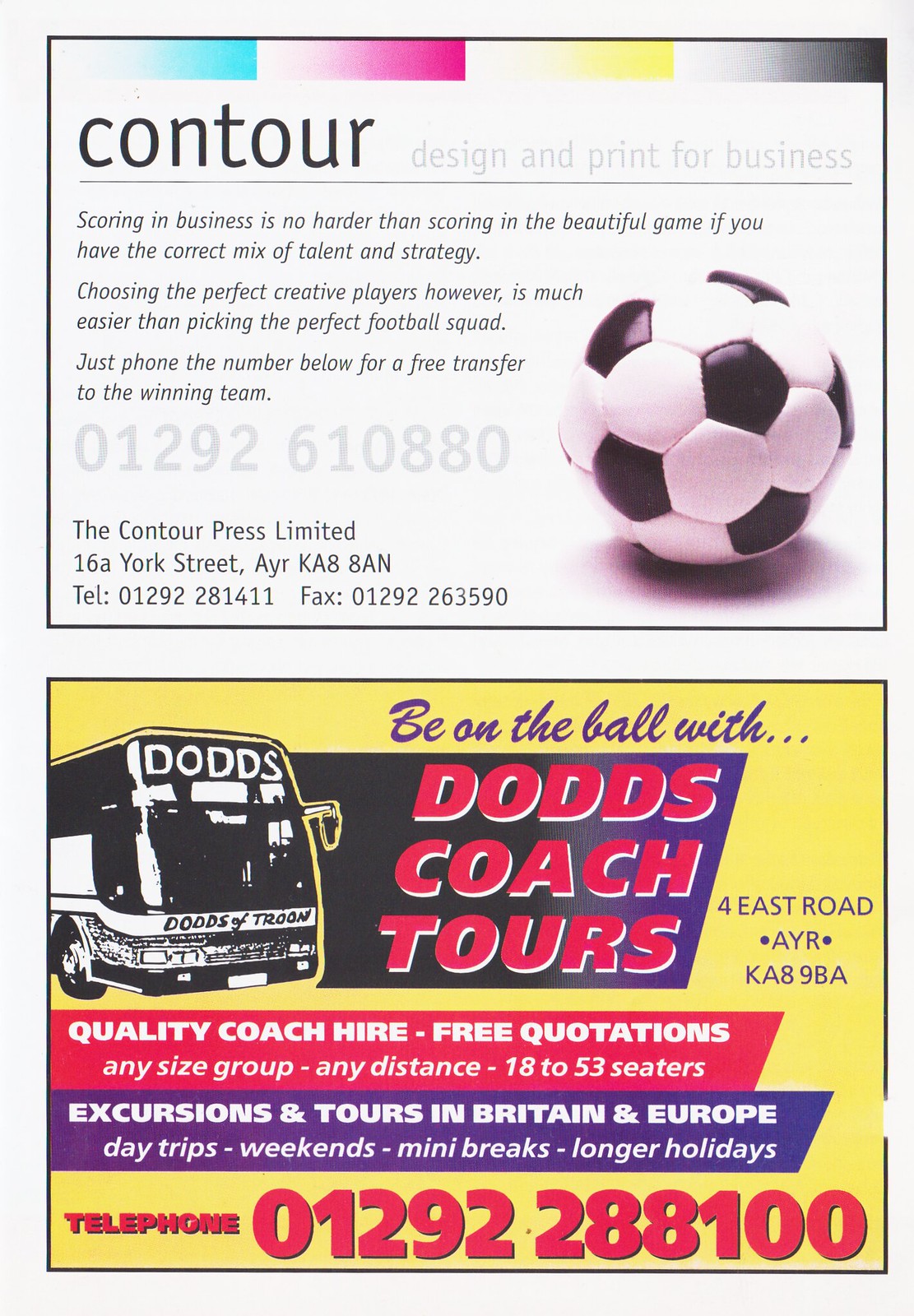The image features two distinct advertisements, each framed by black outlined squares. The top advertisement prominently displays the word "Contour" in black letters beneath a colorful header with four rectangular forms in green, red, yellow, and gray. Subtitled "Design and Print for Business," it includes promotional text suggesting that "choosing the perfect players" in business is as crucial as selecting a football squad, urging viewers to "phone the number below for a free transfer to the winning team." A soccer ball is positioned in the lower right-hand corner, and the ad concludes with the firm’s details: "The Contour Press Limited," its address at 16A York Street, AYR KA88AN, and contact information including a telephone and fax number.

Directly below, the second advertisement showcases "Dodds Coach Tours" with an image of a bus on the left side. Above the company name, the phrase "Be on the ball with" invites potential customers. The ad highlights their services in a red box, listing "Quality coach hire, free quotations, any size group, any distance, 18 to 53 seaters." Below this, another purple box advertises "Excursions and tours in Britain and Europe" including day trips, weekends, mini-breaks, and longer holidays. The company's address, "4 East Road, AYR KA89BA," and the telephone number "01292 288100," rendered in prominent red lettering, finalize the detailed information.